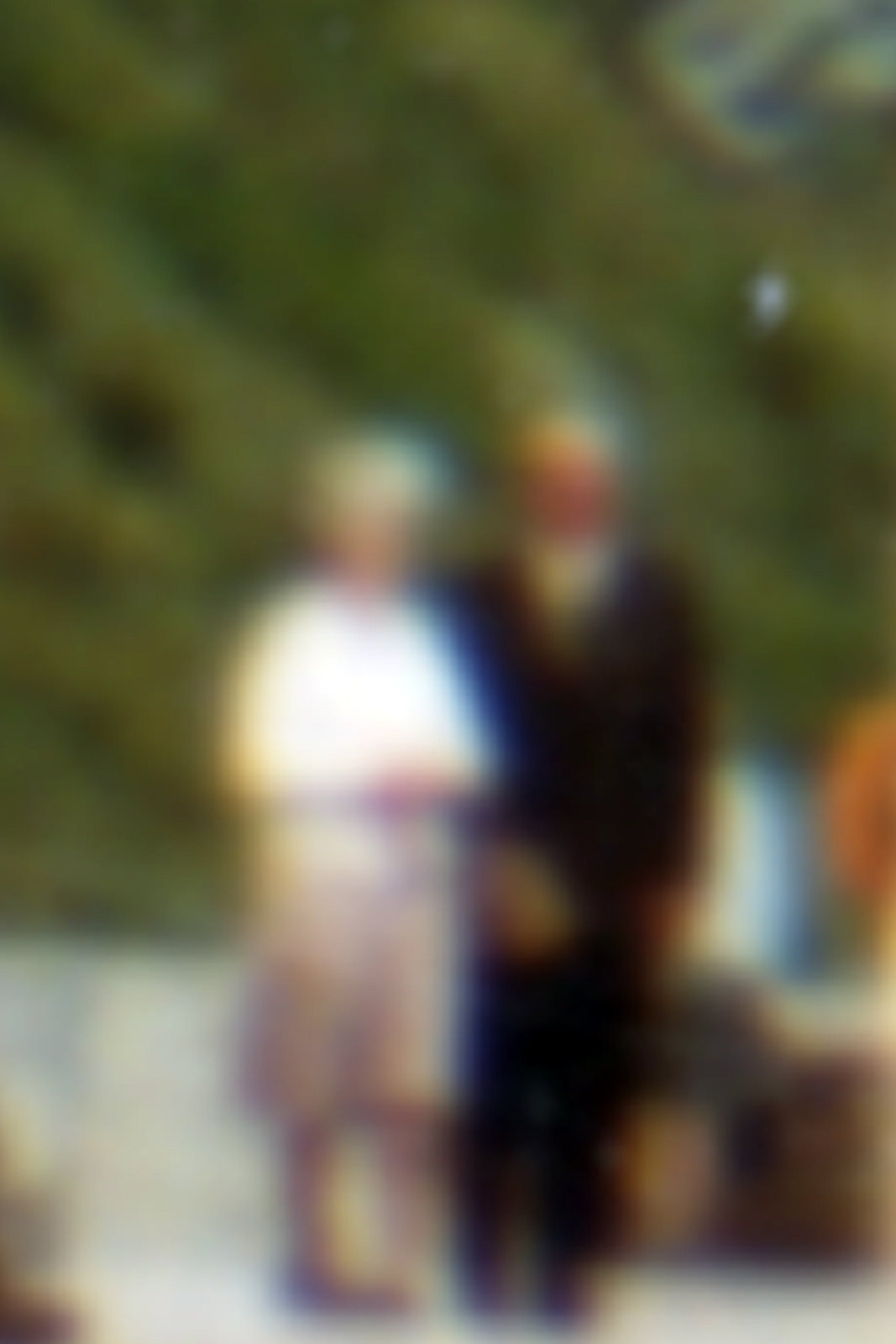This vertically rectangular photograph is extremely blurry and distorted, depicting an elderly couple standing side by side. The woman on the left has light-colored or white hair and is wearing a light-colored, glowing top paired with a somewhat pinkish skirt. The man on the right, who seems to be bald or have light-colored hair, is clad in a black suit with a white shirt. Both appear to have fair skin tones, though the photo's blur makes it difficult to discern details clearly. Behind them, the background features indistinct greenery, suggesting an outdoor setting. The image is notably unclear, with various blocky shapes in shades of brown, white, and orange visible amidst the greenery.